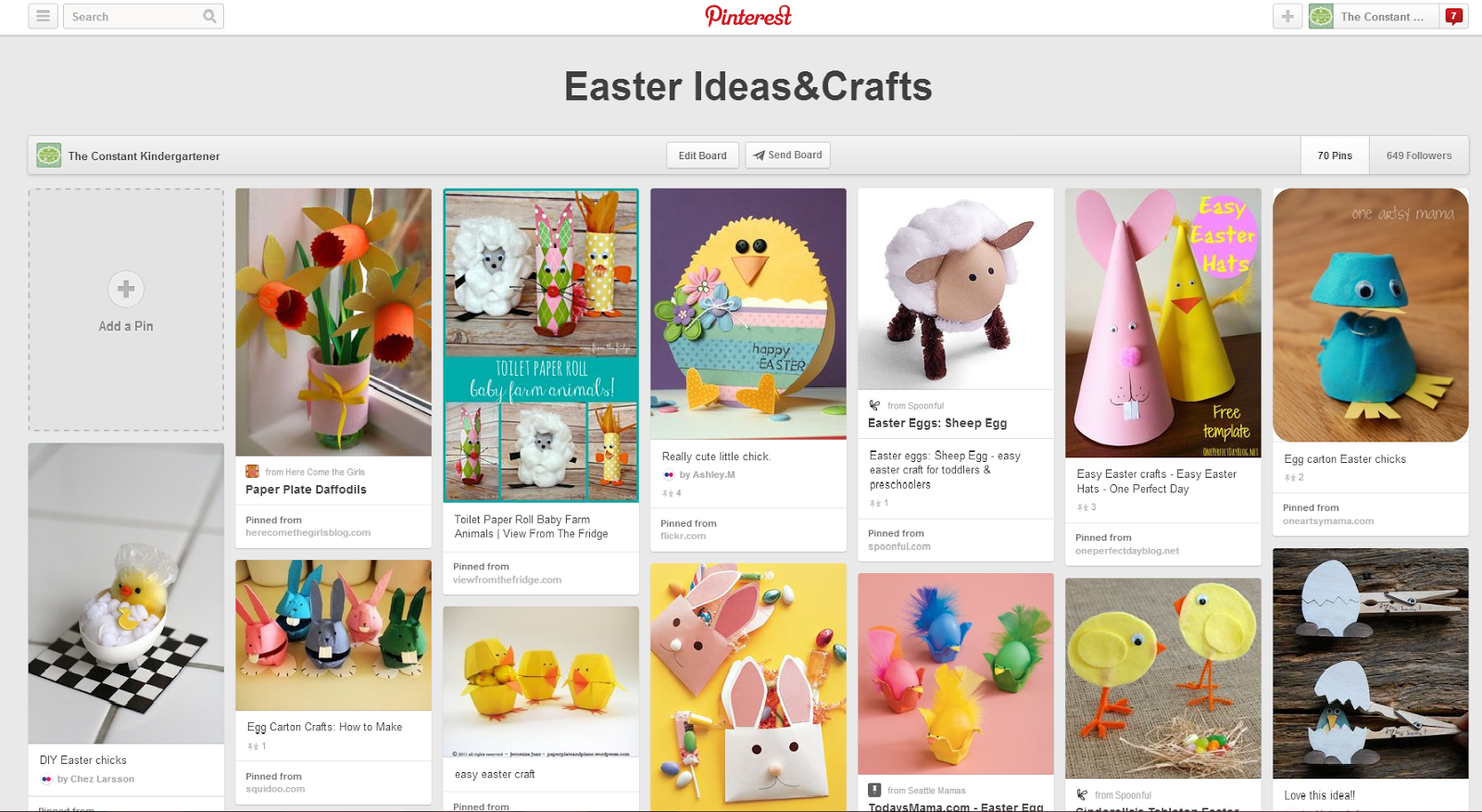This image is a screenshot of the Pinterest website. At the very top, the red Pinterest logo is prominently displayed. Just below the logo, a grey bar features the text "Easter Ideas and Crafts." Below this, there are a few menu bars, which appear to be search bars, although they are somewhat difficult to read. The main section of the page showcases Pinterest's characteristic tiled format, displaying numerous images. Each tile contains a photograph that is Easter-themed, including decorated Easter eggs, handmade chickens, bunnies, and other festive crafts.